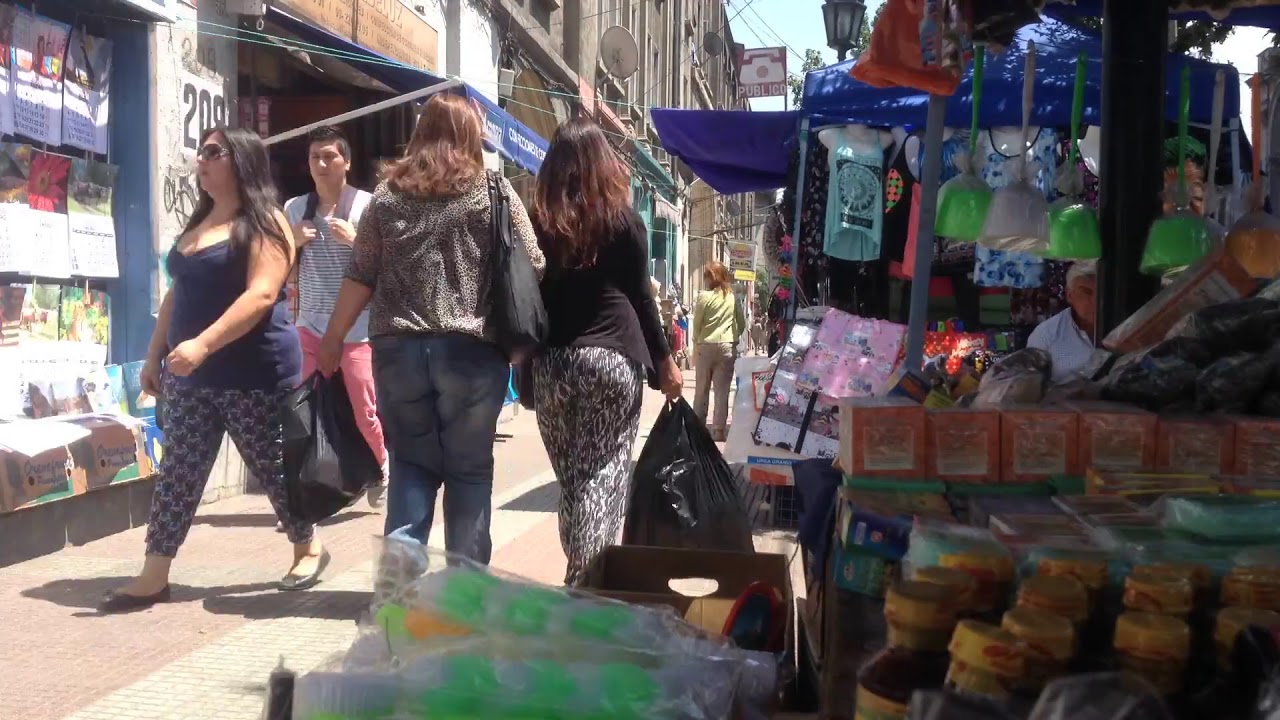This photograph captures a bustling, sunlit urban sidewalk market scene. Dominating the foreground are market stalls laden with colorful products, including sauces with yellow caps, vibrant dusters in mint green and pastel pink, and various jars and boxes in hues of pink and green. In the center, a prominent booth displays many food items. To the left, a building with a large display window and awning has short posters and numbers "209" or "208" visible above a woman's head.

Four adults are featured prominently in the image: two walking towards the camera and two walking away. Closest to the camera on the left, a woman with long dark hair in a black tank top, gray and black-patterned leggings, and slip-in black shoes strides past. Trailing her is a man of Asian descent with a white striped shirt and a backpack slung over his shoulder. On the right side, two women walk away from the camera; one with long light brown hair clad in a loose grayish-green t-shirt and blue jeans, and the other with long dark hair, a black long-sleeve shirt, and light gray patterned pants. Rightmost in the image, a woman carries what appears to be a black trash can.

In the background, more details emerge, including a woman with reddish hair in a light green top, gazing towards the shops. Above the street, the signage reads "PUBLICO," and there’s a satellite dish on the wall, with a lamp post visible in the mid-right section. Bright sunlight casts sharp shadows, and the lively scene suggests a warm summer day, with everyone donning summer attire.